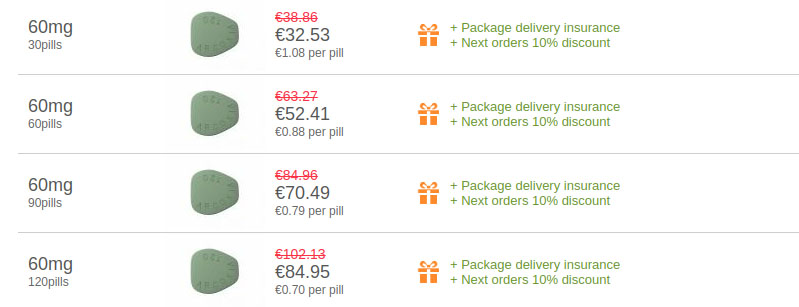The image displays a green tablet that is roughly circular with straight edges, resembling a triangular shape with one end cut off. This 16mg medication is available in four different quantities: 30, 60, 90, and 120 pills. The primary difference across these quantities is the cost, which decreases when purchased in bulk. For instance, the cost per pill for the 30-pill pack is 1.08 Euros, while for the 120-pill pack, it is 0.70 Euros per pill.